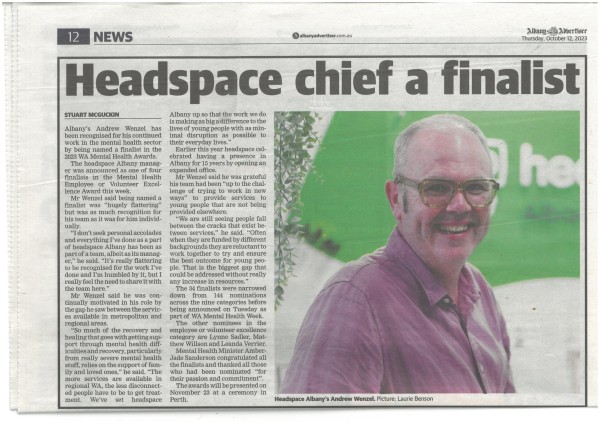The image showcases a newspaper clipping from page 12, dated Thursday, October 12, 2023. The headline reads "Headspace Chief a Finalist." The focal point of the clipping is a photograph of a man wearing a plaid button-down shirt in tan and dark pink hues. He is positioned facing left but turns his head over his right shoulder to directly address the camera with a smile, displaying dimples in both cheeks. The man sports large gray glasses, gray hair with darker sideburns, and stands in front of a partially visible sign that reads "Head..." with a backdrop of tree leaves. The article, which appears slightly yellowed with age, covers his story in detail. At the bottom of the image, a caption credits the photograph, noting: "Headspace Albany's Andrew in a picture taken by Laura Barson."